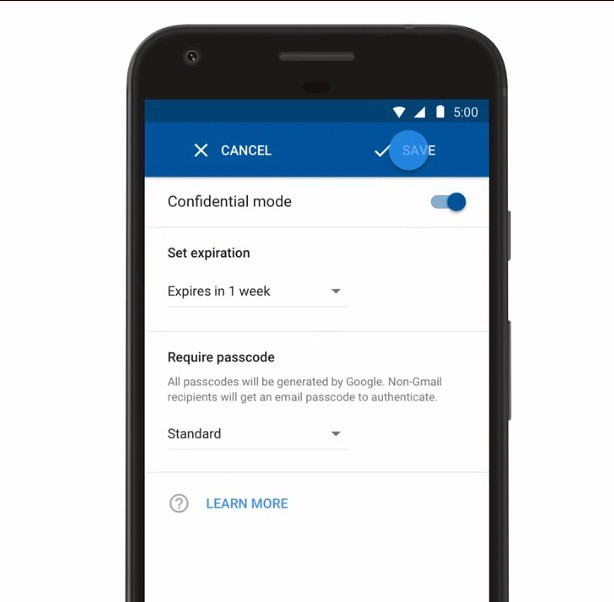This image features an Android phone prominently displayed against a plain white background with a thin black line at the top. The phone, which is black in color and has a front-facing camera, occupies about 80% of the frame; the bottom portion is cut off. The main highlight of the image is the phone's screen, which is explicitly focusing on a "Confidential Mode" settings interface.

The screen displays a top notification bar showing various icons: a fully charged battery symbol, a cell service indicator, a Wi-Fi symbol, and the time, which is set to 5:00. Below the notification bar, the interface shows a horizontal section with a "Cancel" button on the left and a "Save" button on the right. The "Save" button is highlighted in a blue circle with the word "Save" prominently displayed inside it.

Further down, the screen reads "Confidential Mode," indicating that it is currently turned on. Additional details provided include the expiration setting, which is configured to "Expire in one week," and several security notes: "Requires passcode," "All passcodes will be generated by Google," and "Non-Gmail recipients will get an email passcode to authenticate."

Overall, the image effectively focuses on illustrating the details of the "Confidential Mode" settings available on Android devices.